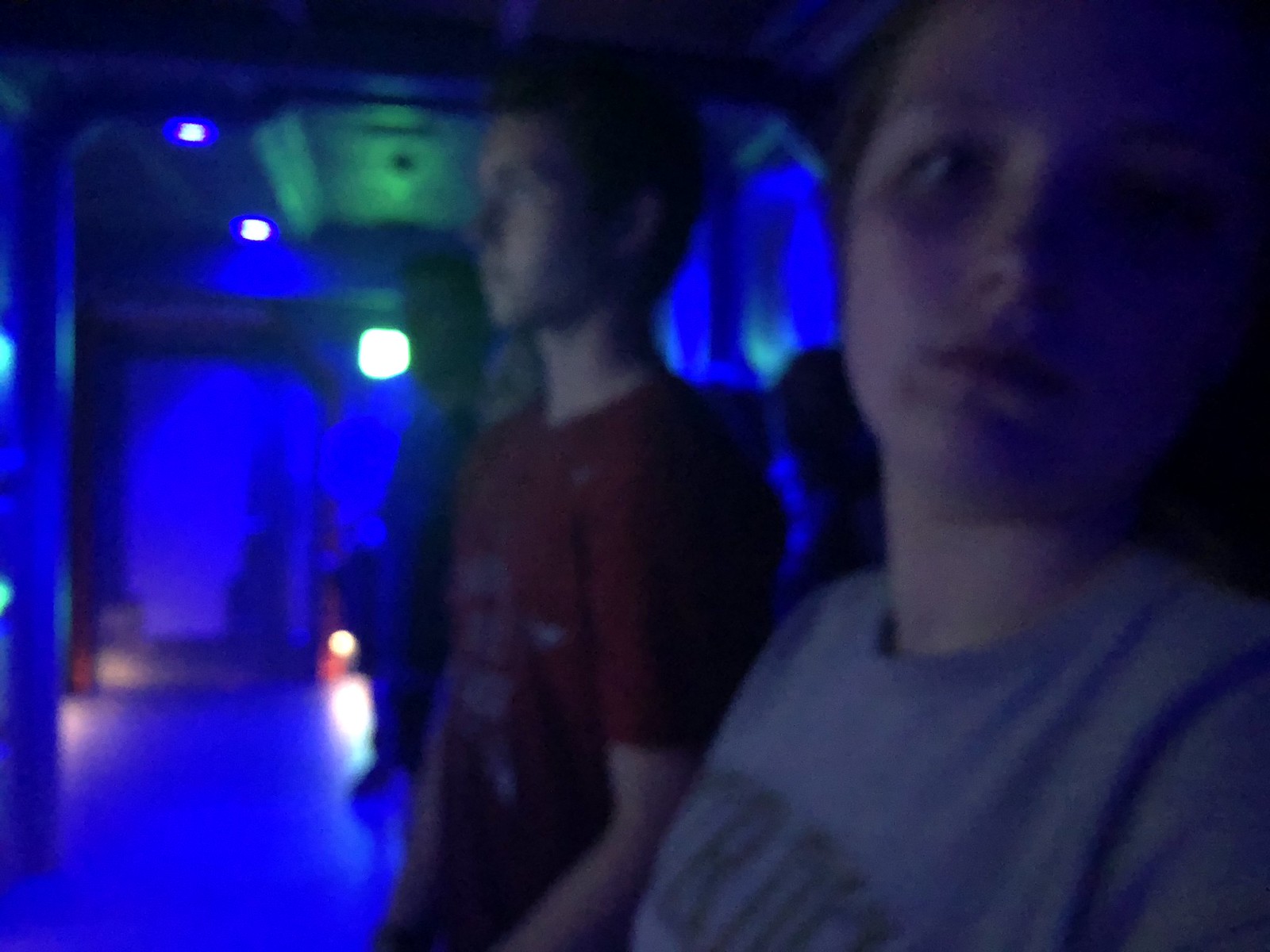The image is a horizontally oriented, blurry selfie taken indoors, likely in a pre-show room of an amusement park ride. The room is bathed in a vivid blue luminescent light, creating a striking blue glow on the walls, ceiling, and floor. In the foreground, there are two teenagers facing the camera; the girl is on the right side of the image, wearing a gray t-shirt with indiscernible writing on it, and looking into the camera with brunette or possibly red hair. Next to her, on the left, stands a boy in a dark red t-shirt with some graphic, looking straight ahead. Both appear to be white. Lining up behind them are other people, partially visible in the bluish haze. You can make out at least one adult in a blue shirt, though details are obscured either by the lighting or motion blur. The overall scene is characterized by its striking blue LED illumination, conveying the ambiance of an immersive, futuristic waiting area.